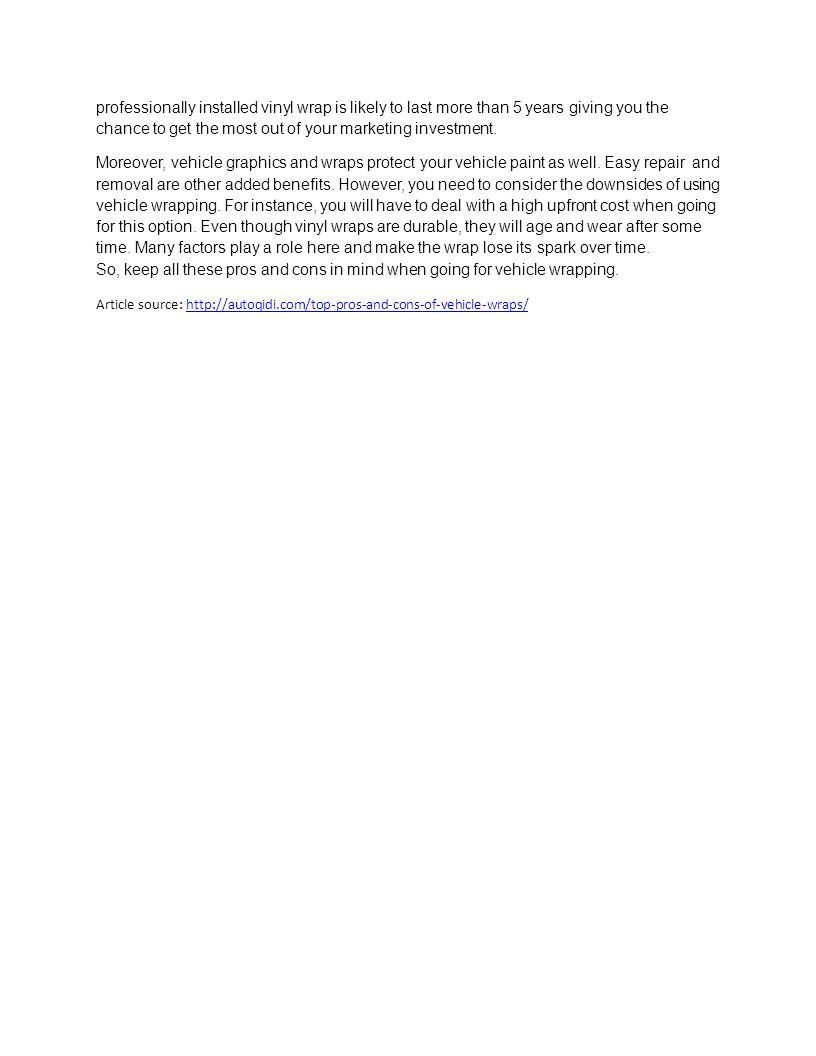A professionally installed vinyl wrap can significantly benefit your vehicle and marketing efforts. According to an article on AutoQidi.com, such wraps can last over five years, maximizing your marketing investment. Furthermore, vehicle graphics and wraps protect your vehicle's paint and offer additional benefits such as safe repair and removal. However, there are downsides to consider, including the high upfront cost and the fact that, despite their durability, vinyl wraps will eventually age and wear. Various factors can diminish their appearance over time. The article encourages weighing both pros and cons before deciding on vehicle wrapping. For more details, you can access the full article at: [Source: AutoQidi - Top Pros and Cons of Vehicle Wraps](http://autoqidi.com/top-prose-and-cons-of-vehicle-wraps).